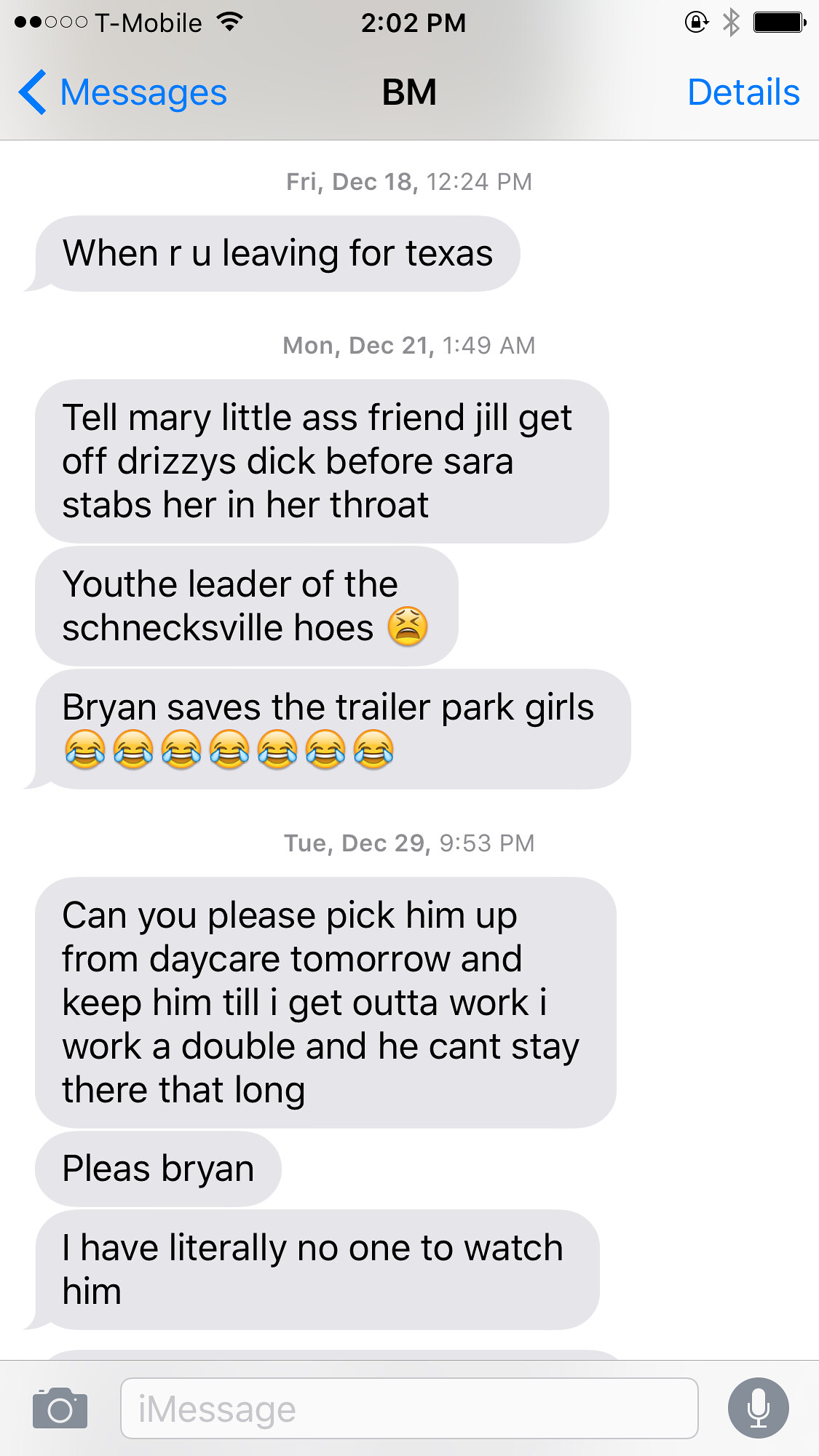The image is a detailed screenshot of text messages from a T-Mobile phone, displaying several key pieces of information. In the top left corner, "T-Mobile" is shown with a wireless connectivity logo, along with the time "2:02 PM", a battery icon, and a Bluetooth logo on the upper right. The screen title "Messages" is displayed beneath this, indicating the texting interface. 

The messages appear to be associated with the initials "BM" and cover various dates in December, starting with one timestamped Friday, December 18th at 12:24 PM. The conversation includes a series of text bubbles, all aligned on the left side, and primarily in light gray against a white background. 

The content of the messages includes inquiries and comments such as "When are you leaving for Texas?" and more vulgar exchanges, mentioning "Tell Mary, little ass friend," and "Jill, get off Drizzy's dick before Sarah stabs her in the throat." Further messages indicate personal requests and interactions, such as "can you please pick him up from daycare tomorrow and keep him till I get out of work?" followed by pleas like, "Please Brian," and "I have literally no one to watch him." 

Emojis with smiley faces and crying expressions are intermittently used to convey emotions. Near the bottom left of the screen, icons are shown for sending photos and a microphone, typically used for voice messages.